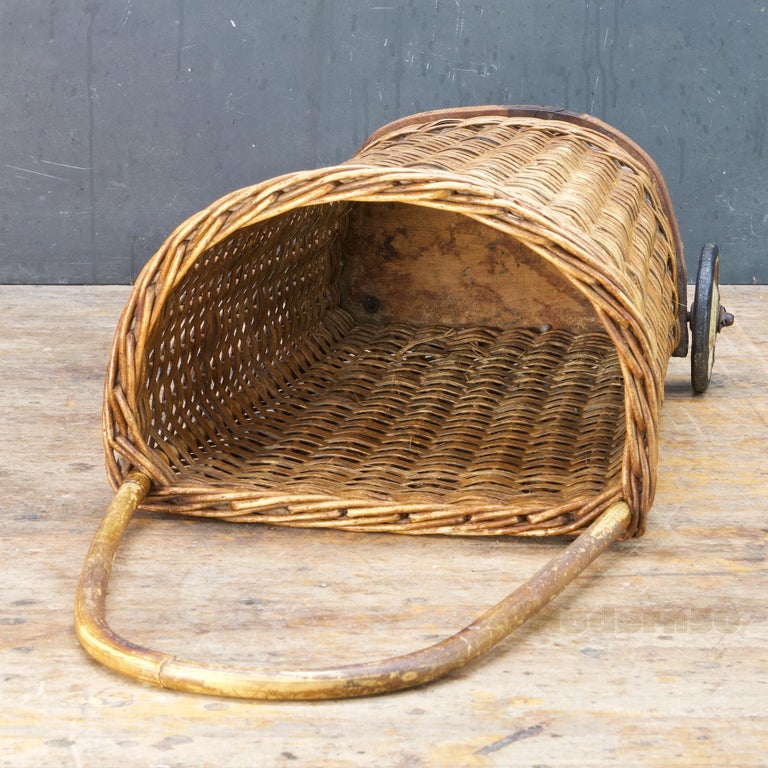The photograph captures a well-worn, wheeled rattan basket lying on its side against a wooden floor and a gray wall. The basket, which resembles a laundry hamper or a rustic grocery shopping cart, features an old, discolored curved handle facing the viewer. Its light golden woven rattan appears aged and heavily used, with indications of significant wear. The bottom of the basket, made of stained plywood, further emphasizes its vintage condition. One wheel with a black tire is visible at the upper right-hand side of the basket, suggesting that the handle is designed for pulling the basket. The entire scene, including the striated, multi-colored beige floor and the dark gray background, adds to the aged, rustic charm of the basket.